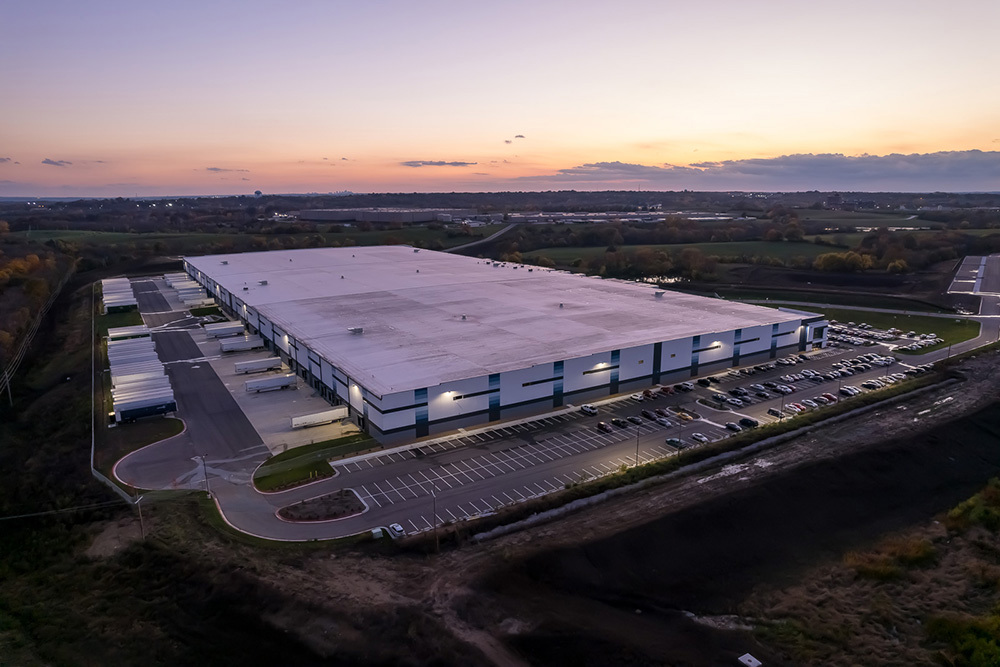The image captures an aerial drone shot of a massive, white warehouse facility, characterized by its flat, table-like structure and expansive surrounding. The warehouse, large enough to resemble a small town, features prominent blue and green stripes on its sides. The left side of the building is lined with semi-trailers and docks, indicating loading and unloading areas. In the foreground is a large parking lot, filled with tiny cars that highlight the scale of the facility, presumably belonging to the employees. 

The scene extends into a rural setting, with green and brown patches of grass and dirt, scattered trees, and distant farmlands. Additional buildings and various houses can be seen sprinkled in the background. The image captures a sky tinged with the oranges and soft light of a setting sun, dotted with clouds, adding a sense of tranquility to the scene. The weather appears to be fair, enhancing the clarity and breadth of the photograph. 

Overall, the composition of the image emphasizes the sheer size of the warehouse and its integration into a rural landscape, possibly hinting at it being a large hub, maybe an Amazon facility, set amid expansive natural surroundings.